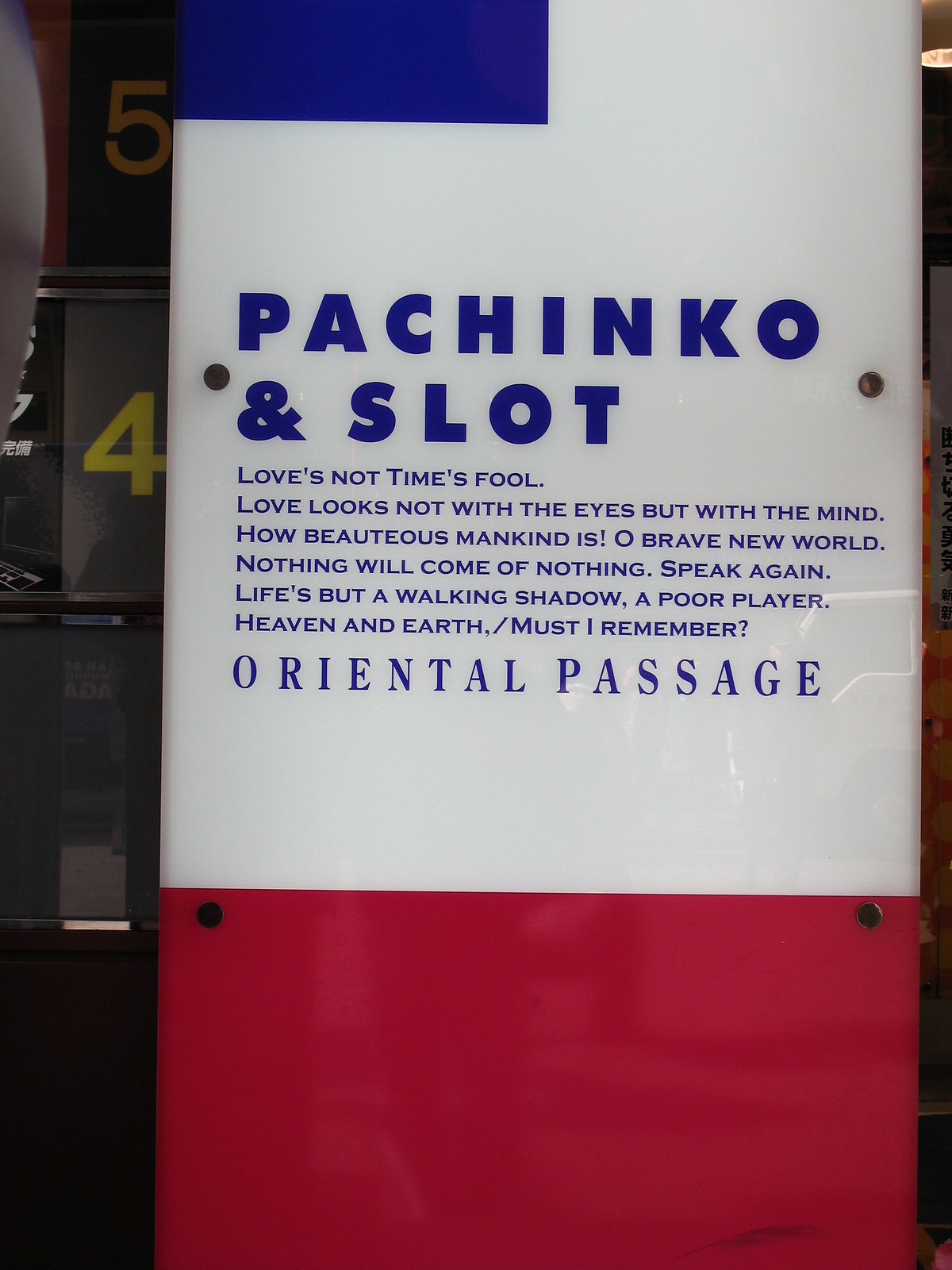The image features a white sign that appears to be securely fastened with two screws on each side. Below the white section, there is a pink area, also affixed with two screws. To the left of the sign, we see the yellow numbers "5" and "4" against a black background. The sign's top half is primarily white with blue text, prominently displaying in bold, all caps: "Pachinko and Slot." Below this, there is a series of poetic lines also in blue, including: "Love's not time's fool," "Love looks not with the eyes but with the mind," "How beauteous mankind is," "O brave new world," "Nothing will come of nothing," "Speak again," "Life's but a walking shadow," "A poor player," "Heaven and Earth," and "Must I remember." At the bottom of this text block, "Oriental Passage" is written in larger blue letters. The very bottom of the image features a red section, while the lower left corner reveals a brown area behind the sign. The right side of the image shows various indistinct objects.